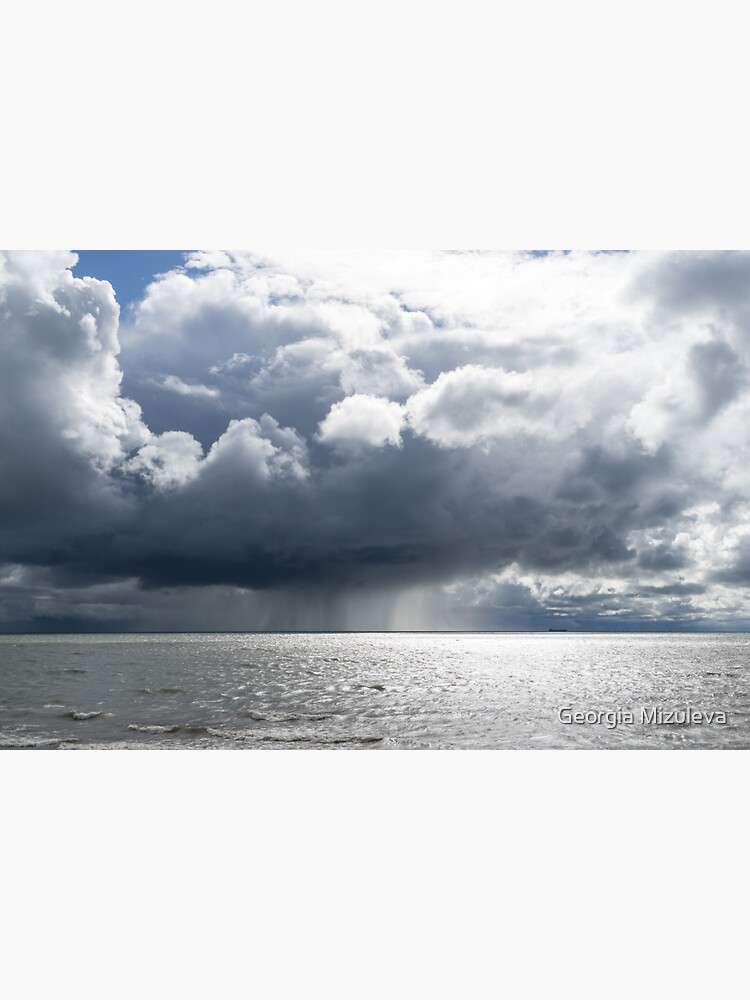This is a color photograph taken outdoors in landscape orientation, depicting a dramatic storm forming over the ocean. The scene captures a contrast between the serene water, which occupies the lower quarter of the image and is still except for small white ripples, and the ominous sky above. The sky features a mix of blue and towering masses of fluffy cumulus clouds, transitioning to darker, heavily laden storm clouds at the bottom. These dark clouds hang low over the horizon, almost touching the ocean’s surface, with visible streaks of rain pouring down. To the left side, the ocean appears shadowed while the right side reflects intense sunlight that illuminates the upper parts of the clouds, emphasizing their white cumulus edges against the dark underside. The overall cloud cover is dense, suggesting turbulent weather, with potential hurricane activity evident in a central funnel-like formation transferring energy between the clouds and the ocean. The image is framed with a thick white border at the top and bottom, and there is a credit in white text in the bottom right corner reading "Georgia Missou-leva." The photographic style is representational realism, capturing the dramatic interplay of light and dark in this natural spectacle.